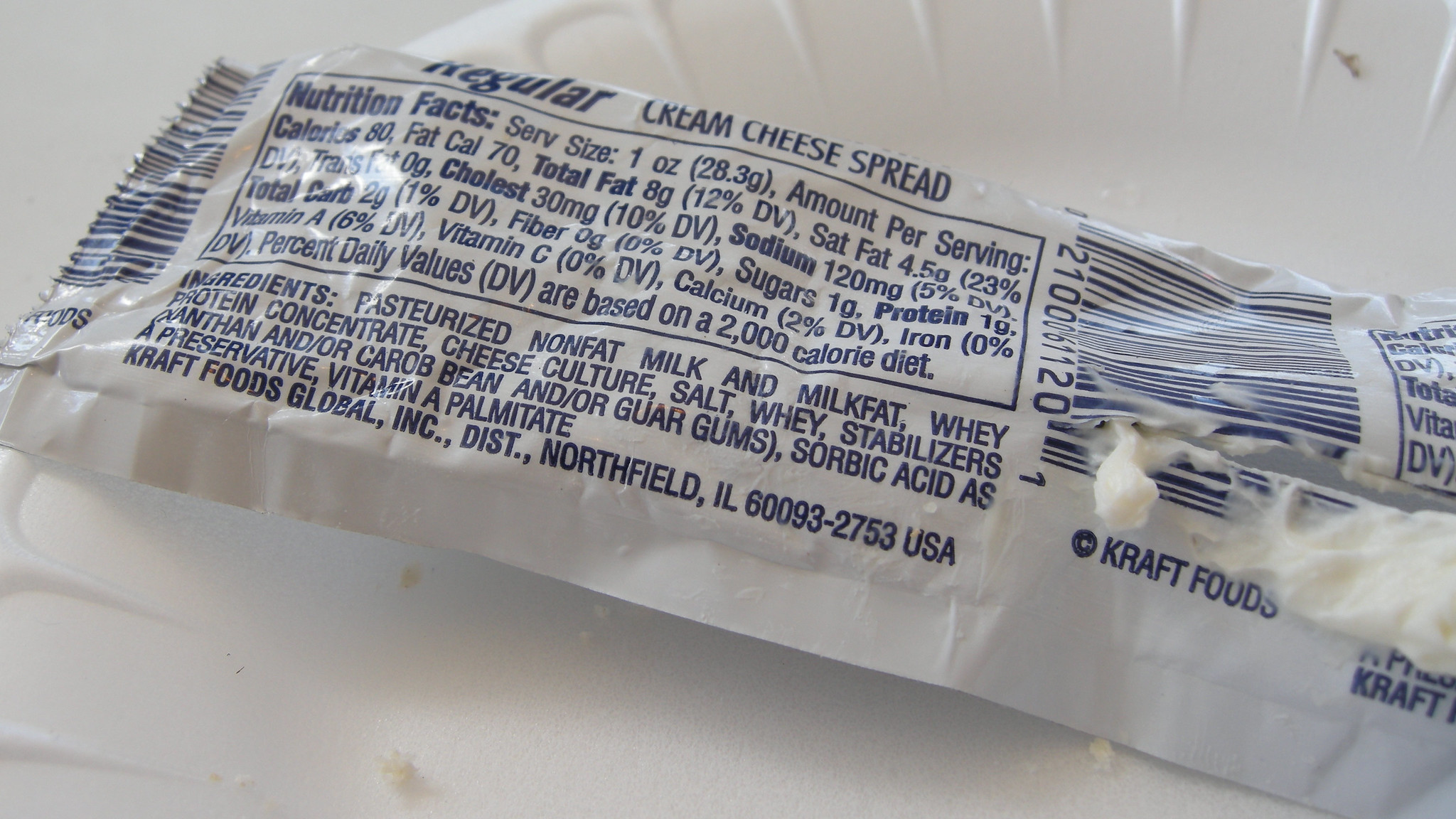This image captures a slightly crumpled white paper wrapper containing food, specifically a regular cream cheese spread. The wrapper displays blue text at the top stating "Regular Cream Cheese Spread." Directly below this, detailed nutritional information and a list of ingredients are printed, adding to the wrapper's informative layout. At the bottom of the wrapper, it notes that the product is distributed by Kraft Foods Global, Inc., located in Northfield, Illinois, with the ZIP code 60093-2753, USA. Additionally, a blue Kraft Foods stamp is visible to the right. The wrapper is placed on a ridged disposable plate, likely made of styrofoam or plastic, and the entire setup rests on a clean white surface.